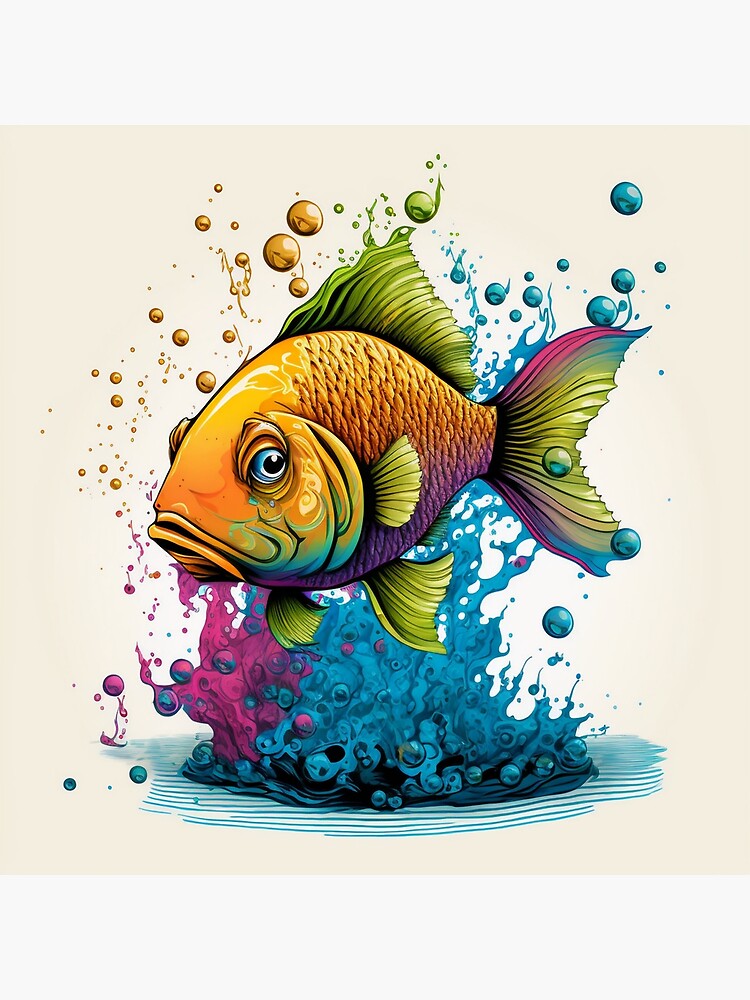This digital artwork depicts a vividly colored fish, likely a goldfish, floating in an airy, ethereal environment. The fish’s main body transitions from a golden hue at the front to a gradient of orange and purple towards the bottom. Its top fin is distinctively lime green, while the bottom fins share the same bright lime green color. The dorsal fin showcases an array of colors, including pink, blue, green, and purple. Surrounding the fish, the background is adorned with bright pink and blue hues that resemble bubbles rising up in a smoke-like manner, transitioning into shades of orange, green, and blue towards the top. Light blue lines at the base suggest the flow of water, perhaps indicating the fish has just splashed out. The entire scene blends elements of undersea life with a dreamlike, atmospheric quality, capturing the eye with its bright, tropical palette.